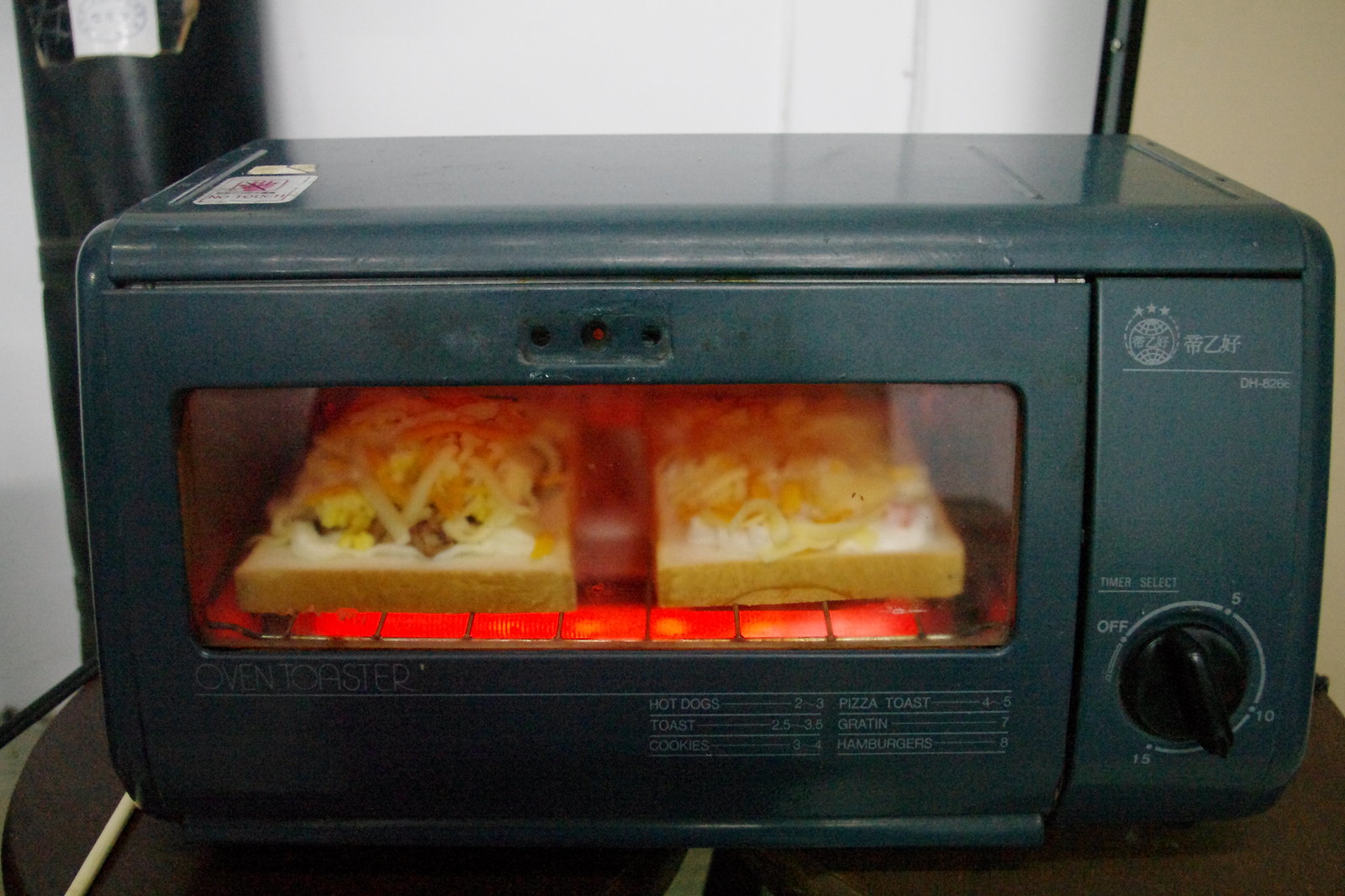This is a detailed color photograph of a dark grey toaster oven in what appears to be a dorm room or small apartment. The toaster oven occupies the majority of the frame, set against a white surface behind it and a beige surface to its right. To the left, there's a black column with an unreadable white sign on top. The oven sits on a brown floor covering.

The oven's front features a rectangular window through which we can clearly see it's in operation, with the red heating element glowing inside. The window reveals four slices of bread, some topped with cheese and possibly other toppings, being toasted. At the top of the oven above the glass, there are three small holes. 

On the right side of the oven, there's a dial with some unreadable white writing above it. Underneath the window to the far right, there's more small, unreadable text arranged in two columns. The top left corner of the oven sports a white sticker with a red logo or object in the middle.

The device is equipped with a basic thermostat control, and the door opens to the side. Despite some of the writing being difficult to read, it's noted that the toaster oven is versatile, supposedly suitable for making hot dogs, toast, cookies, pizza, hamburgers, and more.